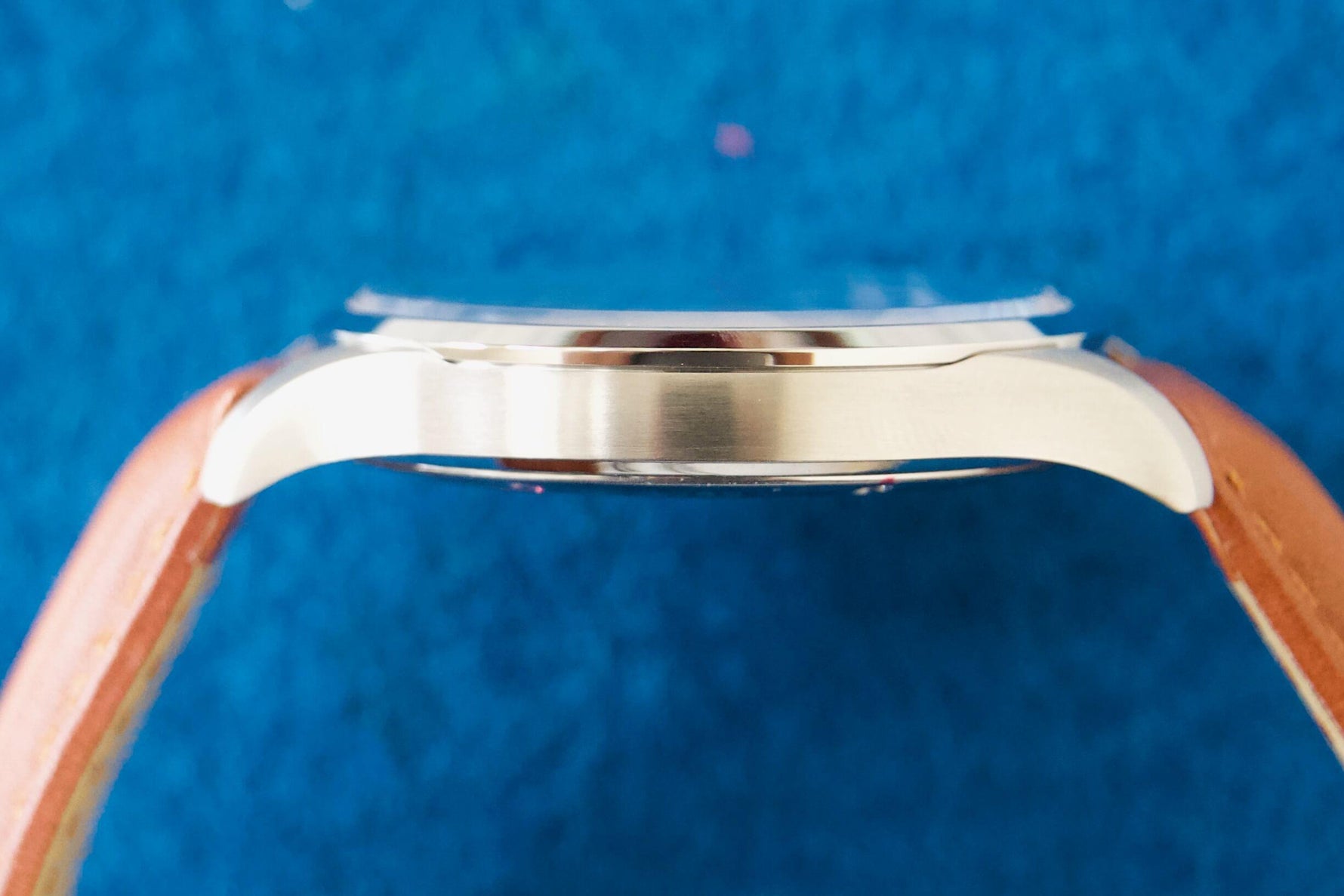The image depicts a side view of a watch set against a blurred, textured blue background that resembles stucco. The watch features thick, diagonal straps extending from both corners of the frame, likely the bands, which are a brownish tan color. At the center of the image is a circular silver component with a reflective surface that mirrors the background's blue hue. The silver centerpiece has a distinctive design, including a rectangular curved shape and a smaller circle within it. The photograph captures the watch from an angle that does not reveal the face but highlights the side profile and the complete structure of the watch.